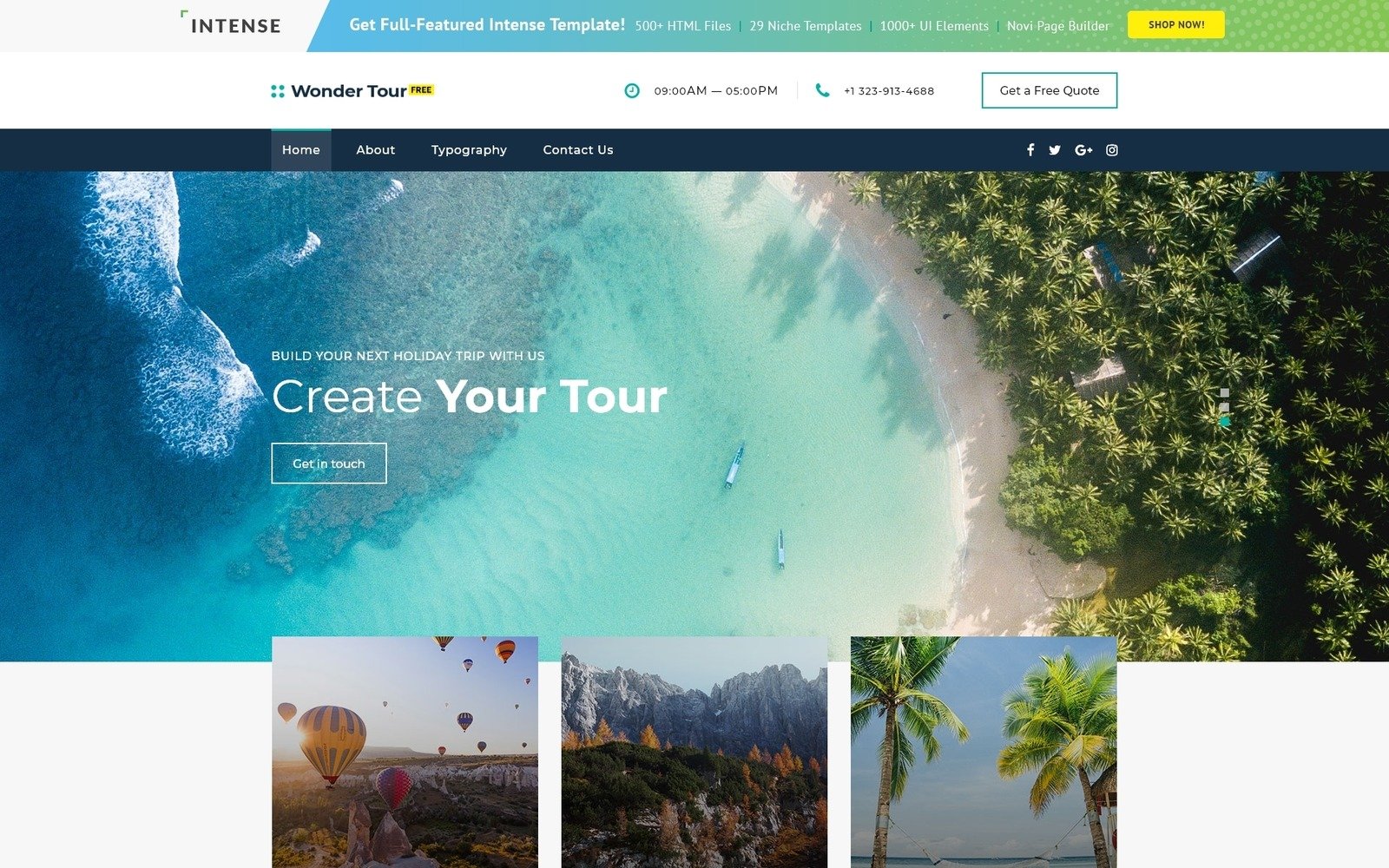Here's a revised and detailed caption for the image:

---

The image is a promotional banner extracted from a website featuring a monochromatic teal-to-green color scheme at the top. Prominent text headings include "Intents", followed by bold statements: "Get Full Featured Intents Template", "500+ HTML Files", "29 Niche Templates", "1,000+ UI Elements", and "Novi Page Builder". Towards the end, there is a conspicuous yellow rectangle with black text stating "Shop Now".

Below this header, another segment labeled "Wonder Tour" indicates the business's operational hours (9 a.m. to 5 p.m.), phone number, and a box encouraging visitors to "Get a Free Quote". The central portion of the banner displays a captivating aerial photograph of a coastal, beachy area with palm trees to the right and small boats drifting in serene teal waters. The photo captures streaks of white water, suggesting boat paths.

As you scroll down, the text overlays "Build Your Next Holiday Trip With Us", "Create Your Tour", and "Get In Touch" guide the viewer towards tour creation and contact options. The bottom section of the image features thumbnail pictures of hot air balloons, scenic mountains, and lush palm trees, adding to the adventurous and tropical theme.

---